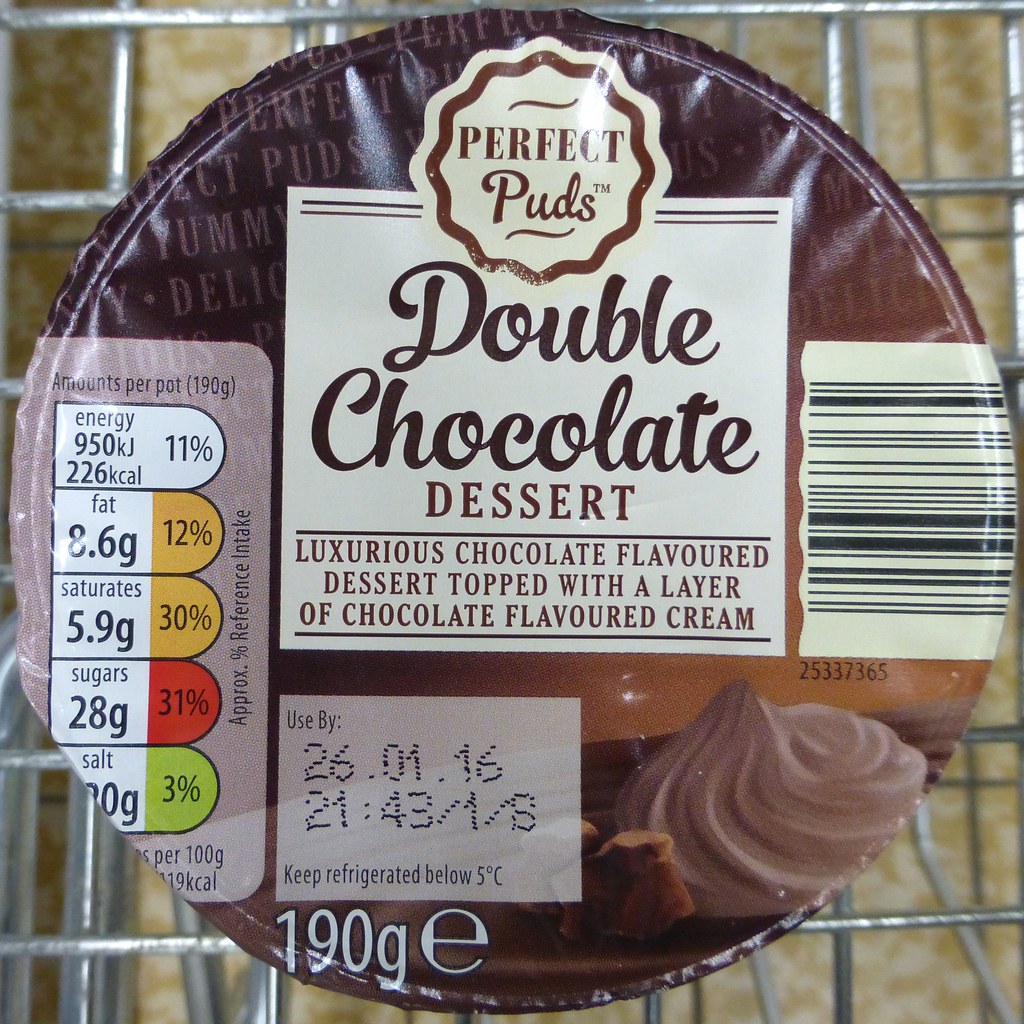This is a highly zoomed-in color photograph of the top of a dessert cup called Perfect Puds, specifically their trademarked Double Chocolate Dessert. The dessert cup is seated on a metal wire rack, presumably in a shopping cart. The label background is primarily brown with lighter brown accents. The top center of the label prominently features the brand name "Perfect Puds" in bold brown letters, below which is the title "Double Chocolate Dessert" in black text. The detailed description reads, “Luxurious Chocolate Flavored Dessert topped with a layer of chocolate flavored cream.” To the right side of the label is a barcode, and beneath it, an image of the dessert showing a layer of chocolate and chocolate-flavored cream. The left side of the label contains nutritional information, indicating values for energy, fat, saturates, sugars, and salt, all listed per 190 grams. The product weighs 190 grams, and the expiration date, printed on a light brown square at the bottom, reads "Use by 26.01.16". Additionally, the label instructs that the dessert should be kept refrigerated below 5 degrees Celsius. The packaging design includes sections of cream-colored boxes containing brown text for better readability of the brand name and product description.